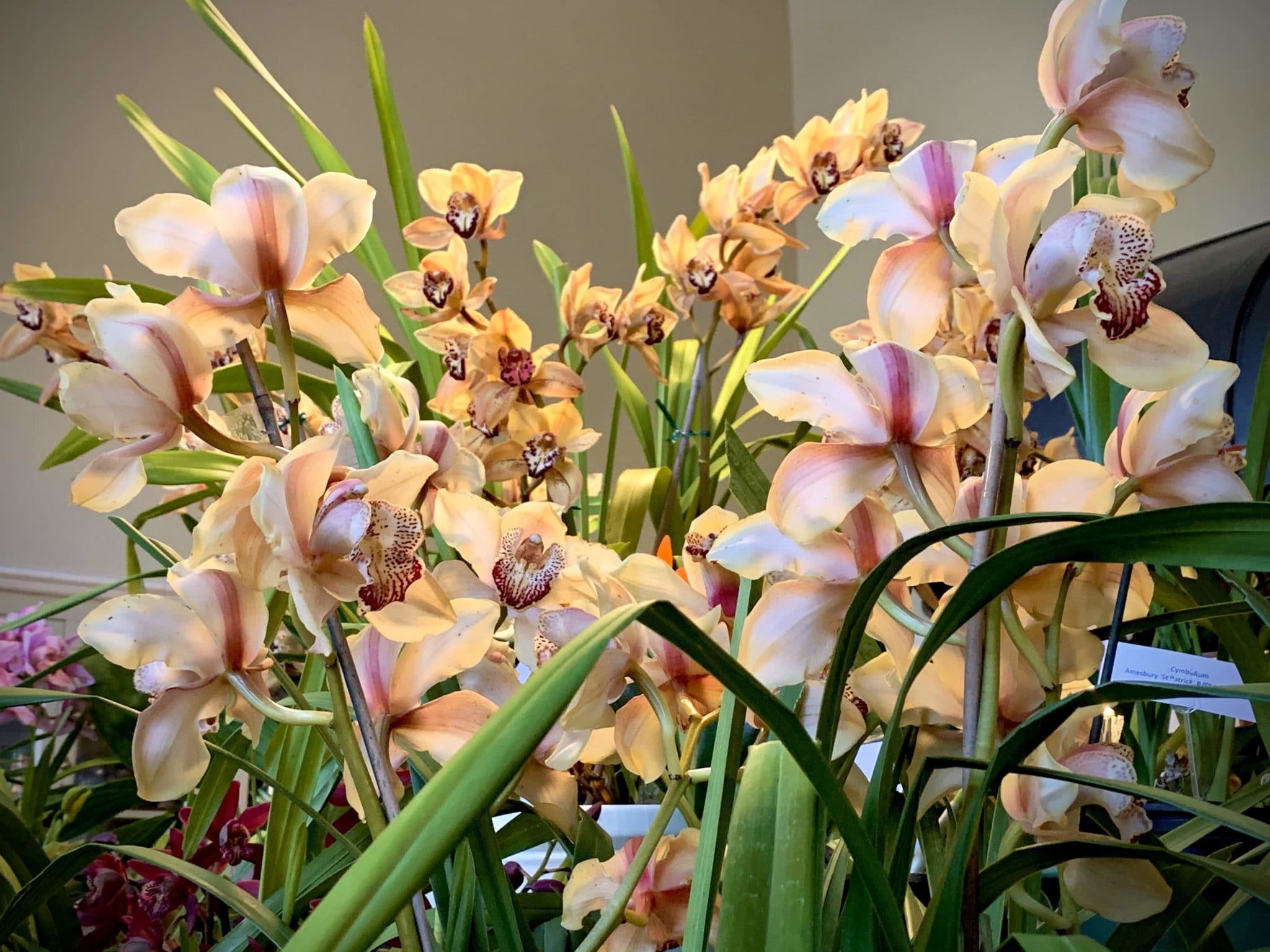This image captures a detailed close-up of a bouquet of clustered flowers dominated by pastel hues, including pink, yellow, beige, cream, and burgundy. The floral arrangement features at least three or four distinct types of flowers, prominently including orchids. Some petals display hints of white, red, and violet, alongside rich green leaves that are both bent and standing upright. The flowers take up the majority of the frame, creating an intricate and layered display. The background is largely out of focus, revealing cream-colored walls that appear to converge in the corner of a room, perhaps accentuated by a dado rail on the left-hand side. There is a small, barely legible white card or tag located at the bottom right, and a possible hint of a flat-screen TV on the wall. The flowers seem to be illuminated by overhead lighting, casting a soft glow over the arrangement.